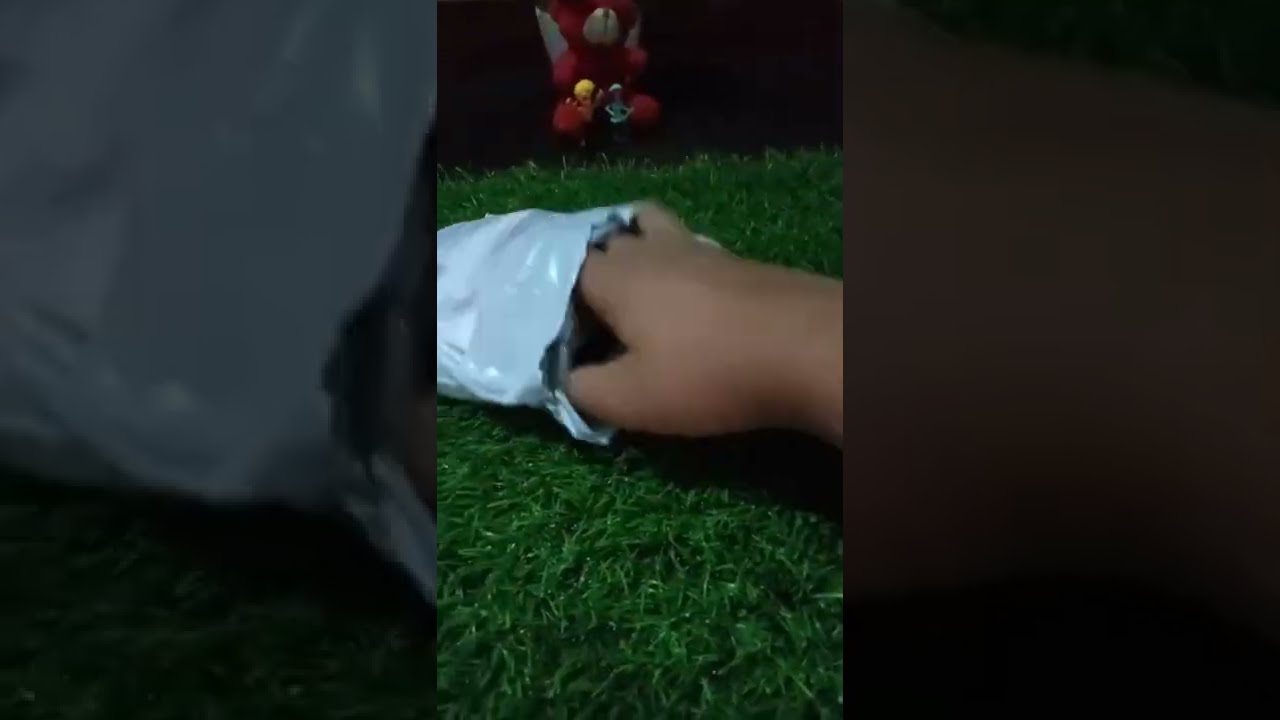The image depicts a small white hand reaching into a white plastic package, reminiscent of an Amazon package, situated on artificial green AstroTurf. The white hand delves into the bag, revealing a gray interior typical of mail packages. Surrounding this central image, an extended background shows the same scene on a larger rectangle, albeit with some areas blurred or darkened. In the distance, part of the image includes a pink or red teddy bear with a white snout, positioned amidst three small figurines: one yellow, one blue or teal, and one that could be interpreted as a screaming banana. The yellow figure sports blond hair with arms raised, while the blue or teal figure, smaller than the others, appears to be playing an instrument. This outdoor setting creates a whimsical and slightly surreal composition, blending the realistic textures of the turf and bag with the imaginative presence of the distant figurines.